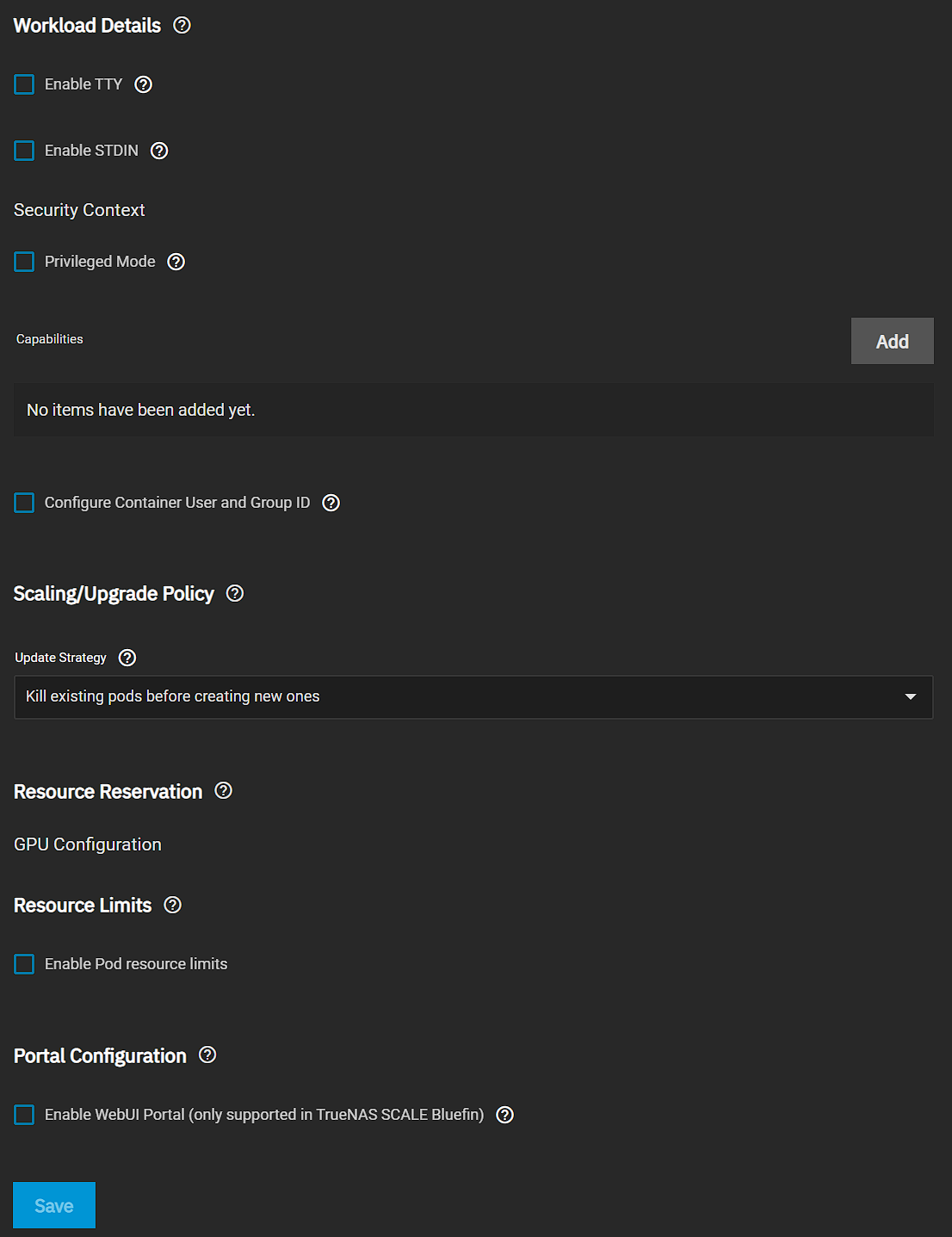The image features a comprehensive administrative dashboard with a primary focus on workload management. The dominant element is a large gray rectangular background titled "Workload Details" at the top. 

Within the rectangle, there are several blue-outlined squares, each accompanied by text and a circle containing icons or symbols, though the specifics of the icons are unclear. These include parameters and options for configuring various aspects of the workload. Key entries among them are:
- "Scaling/Upgrade Policy" with an associated circle containing an icon.
- A segment labeled "Resource Reservation" with the accompanying icon inside a circle.
- "Resource Limits" with a similar formatting, including another icon inside a circle.
- "Postal Configuration" indicated near another circle with an icon.

On the right-hand side of the primary gray rectangle, there is a lighter gray rectangle with the word "Add" prominently displayed in white, suggesting an option to add new configurations or details.

Further down in the interface, a slightly darker gray rectangle appears with text on the left and a downward-pointing arrow on the right, possibly indicating collapsible or expandable information.

At the bottom of the dashboard, various sections are clearly delineated with blue-outlined rectangles, each adjacent to text and a circle with an imbued icon, allowing users to configure additional granular settings.

The "Save" option is highlighted in a blue rectangle at the very bottom of the interface, ensuring user changes can be preserved. 

This detailed layout suggests a rich, interactive tool designed for meticulous workload management and fine-tuning of system parameters.